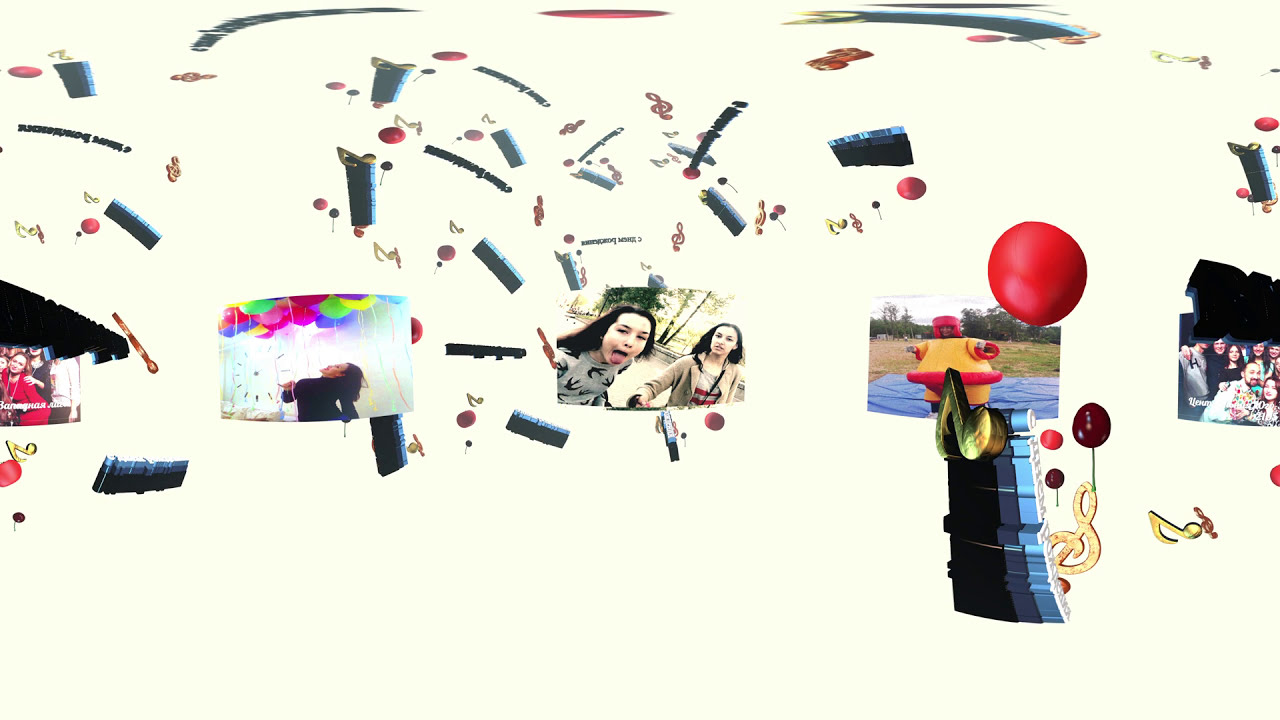This image is a visually cluttered collage set against a tan background, featuring a chaotic mix of random shapes, colors, and designs, prominently centered around five main photos. Among these central photos, the middle one is a selfie of two young individuals, with one girl on the left playfully sticking her tongue out. Flanking this are additional images: to the far left, a girl appears to be in a group, while a woman holding balloons is seen to the immediate left. To the immediate right, a person in an inflatable sumo wrestling suit grabs attention, and another group photo is located on the far right. Scattered throughout the image are various music-related designs, including musical notes and keyboards, along with an assortment of circles and random shapes in multiple colors such as black, dark blue, light blue, yellow, red, pink, purple, green, and white. The overall composition lacks any discernible pattern or text, giving the impression of a personalized montage of memories and miscellaneous elements.